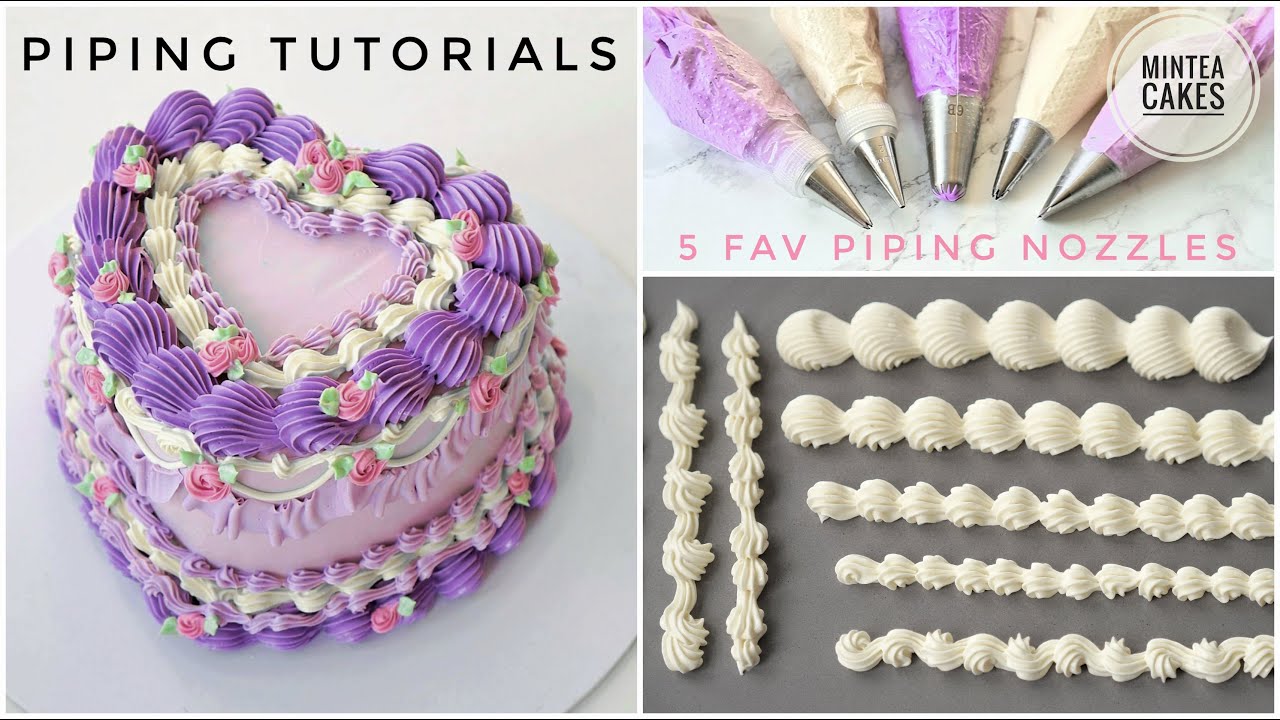This advertisement for a piping tutorials site features a detailed collage of three images, showcasing various aspects of cake decorating. On the left, a heart-shaped cake adorned with elaborate decorations is prominently displayed. The top of this section reads "Piping Tutorials" in black text. The cake itself is extravagantly frosted with purple icing outlining its heart shape and is further embellished with roses connected by green vines. The edges are piped with intricate designs in purple, pink, and yellow, with a ribbon-like pattern encircling the base.

To the upper right, another image highlights five favorite piping nozzles. This image arranges the piping bags in an arch, their nozzles pointed inward, and filled with colorful frostings in shades of purple, white, and pink. Pink text at the bottom of this section reads "Five Fave Piping Nozzles."

The final image at the bottom right showcases different piping techniques on a gray background. Various strings of frosting are displayed, demonstrating the unique designs each nozzle can create, with a mix of long lines and dotted patterns, exemplifying the site’s tutorial offerings.